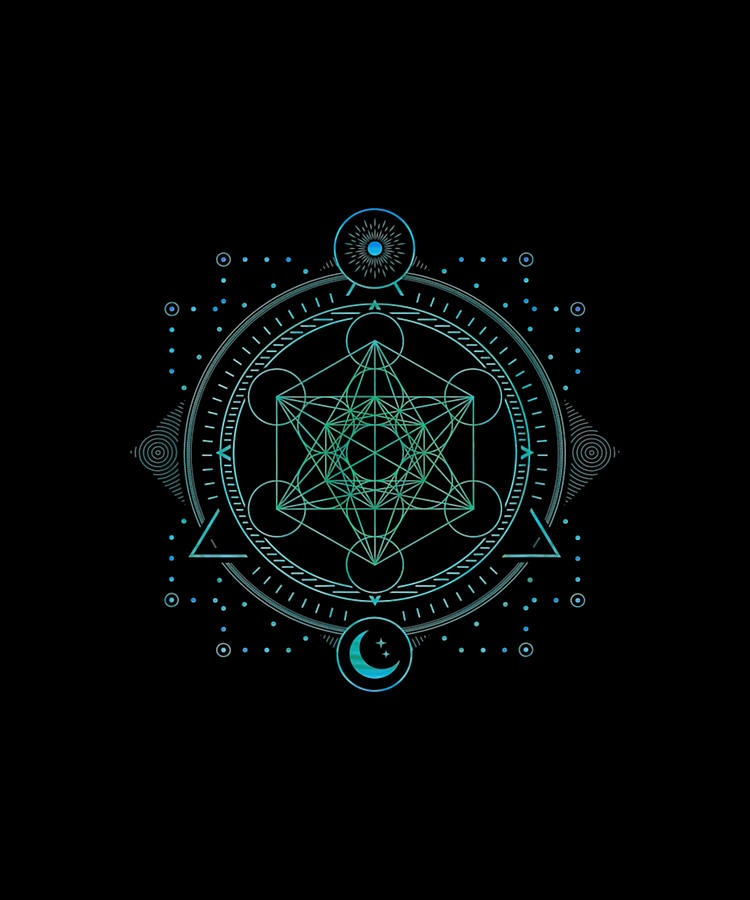The image features an elaborate, abstract celestial design set against a stark black background. Dominated by geometric elements, the centerpiece is a large green circle surrounded by a webbed pattern of lines and circles. This central green circle contains a repeating hexagonal pattern, each comprised of six smaller circles, creating a nested hexagon effect. The color palette primarily includes shades of blue, brown, and green.

Encircling the large central circle, a series of smaller concentric circles in light green and gray are present, adorned with dashed lines and Pac-Man-like dots. At each corner of these patterns, larger dots are encircled, contributing to the overall geometric harmony. Additionally, two triangle shapes with circular designs inside intersect the main design, while two half-triangle shapes are outlined without filling.

At the top of the image, a smaller circle encloses a sun-like pattern. Opposite this, at the very bottom, another smaller circle contains a crescent moon accompanied by two stars. The sides of the central design feature V-shaped patterns and diamond shapes, adding to the intricate detail of the composition. The harmonious blend of straight lines and circular forms gives the artwork a mesmerizing, interconnected appearance.